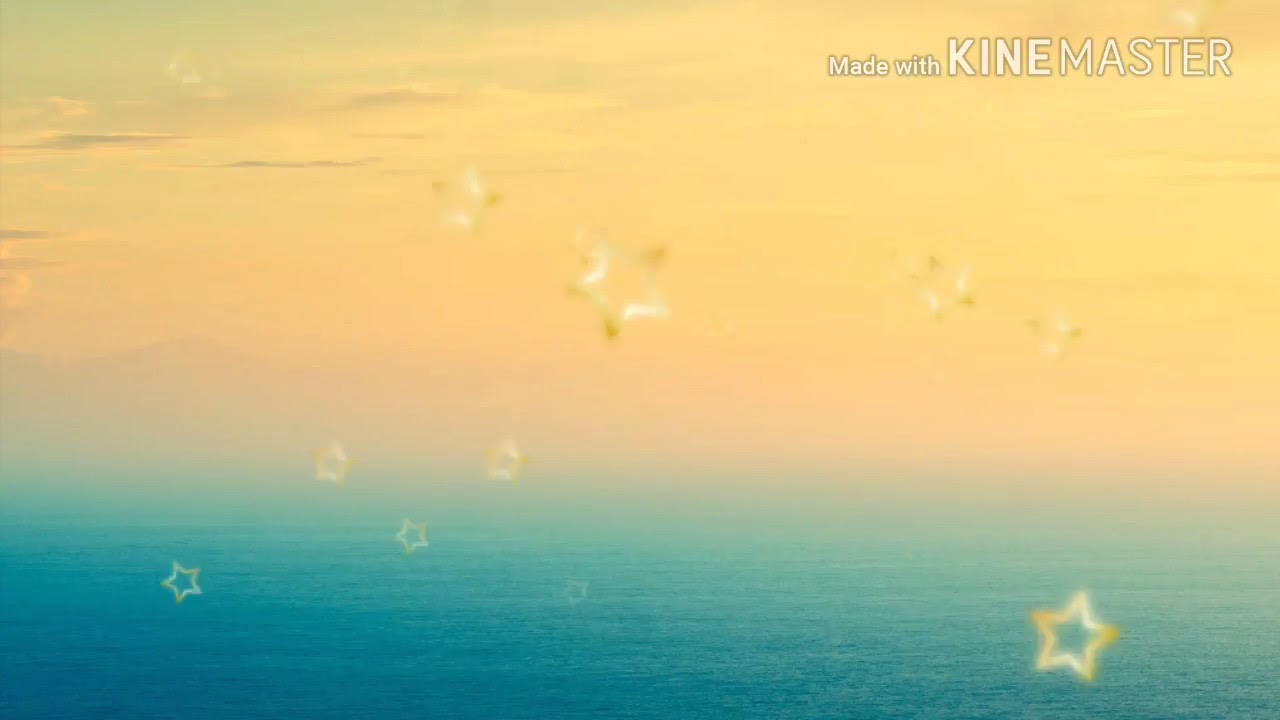The image appears to be a computer-generated artwork created using KineMaster, as indicated by the text "Made with KineMaster" in the top right corner. It showcases a serene, light blue body of water at the bottom, transitioning from a light blue on the right to a darker blue on the left, with a smooth and calm surface. In the background, there are subtle, foggy hills or mountains, adding depth to the scene. Above the horizon, the sky features a blend of peach, yellow, reddish, and pale pink hues, suggesting a sunrise or sunset, with some hazy clouds enhancing the atmosphere.

Superimposed over this tranquil landscape are several three-dimensional, transparent golden stars with white and yellow outlines. These stars, numbering about 11 to 12, are blurred and randomly distributed across the image, adding a whimsical, artistic touch. Although the image is not hyper-realistic, it exudes a poetic and imaginative quality, likely crafted with special software to evoke a dream-like seascape.